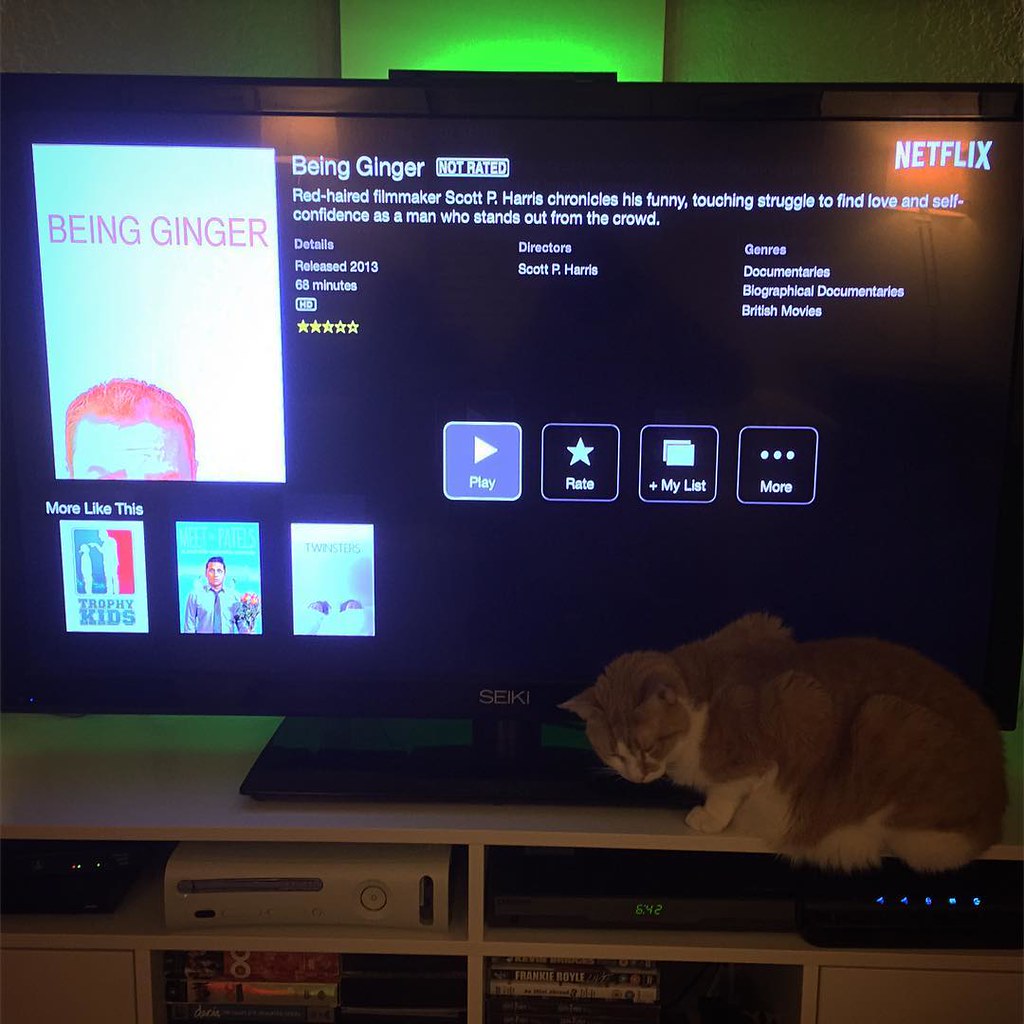In this image, a TV screen is displaying the Netflix interface, specifically showcasing the movie "Being Ginger." In the upper right corner, the word "Netflix" is visible. On the screen's left side, a movie poster for "Being Ginger" is displayed alongside its title and "Not Rated" status. The detailed description reads: "Red-haired filmmaker Scott P. Harris chronicles his funny, touching struggle to find love and self-confidence as a man who stands out from the crowd." The movie was released in 2013, runs for 68 minutes, and has an approximate rating of two and a half stars. Below the description, a set of four options is presented: Play, Rate, My List, and More, the latter marked with three dots.

Further movie details are organized across the screen: directors in the middle, genres—documentaries, biographical documentaries, British movies—on the right. At the bottom, the "More like this" section features three additional movie thumbnails.

The TV, identified as a Seiki model from its brand name in the bottom middle frame, sits on a wooden stand. Below the TV, an Xbox 360, a DVR or Blu-ray player, and some movies and discs are visible. A small cat is perched in the lower right-hand corner of the TV stand, adding a touch of coziness to the scene.